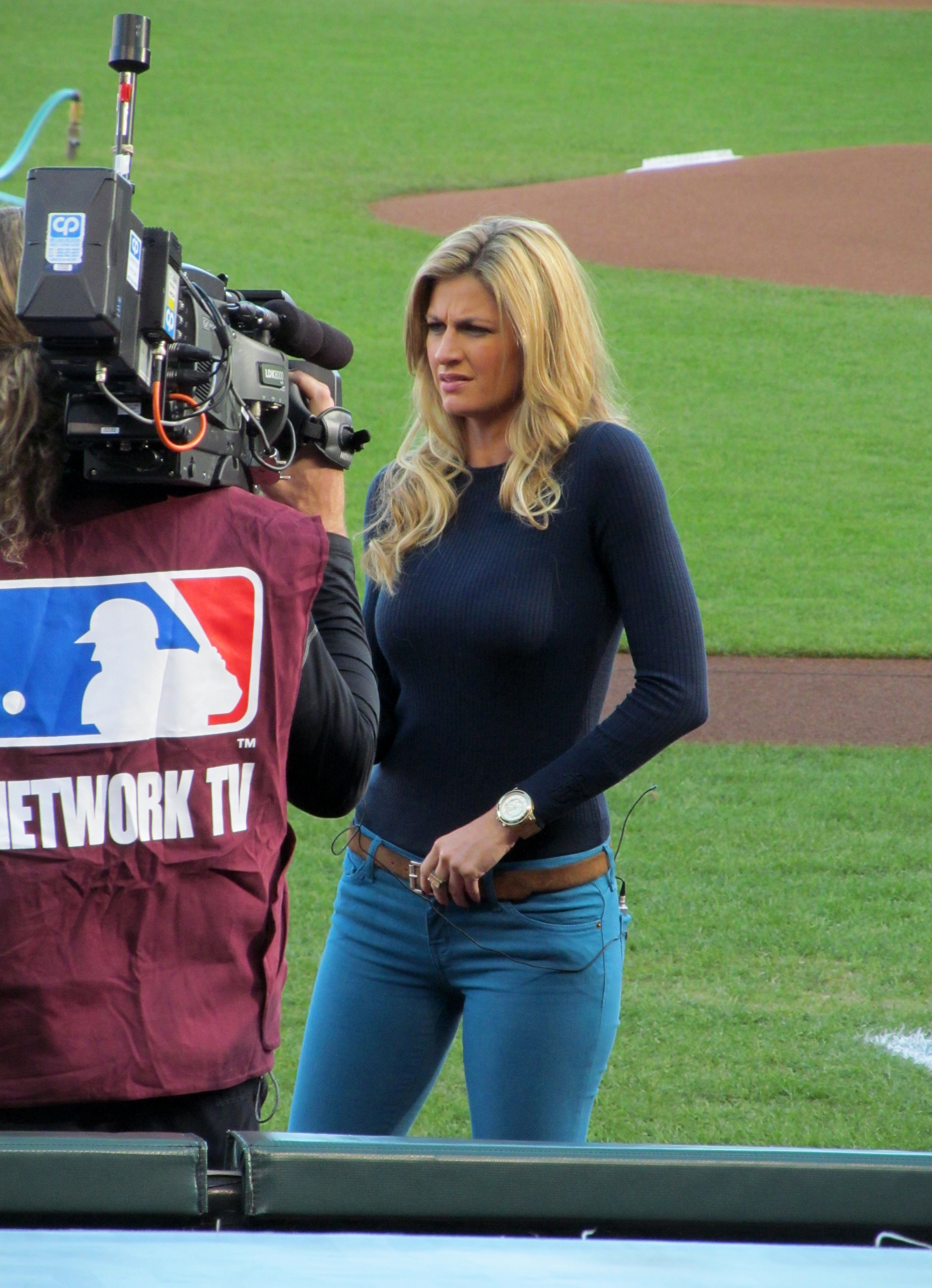This image captures sports journalist Erin Andrews on a baseball field, preparing for a broadcast. She is seen with her blonde hair down, wearing a long-sleeved, dark blue shirt paired with blue jeans and a brown belt. Erin appears focused and possibly unsettled as she looks off to the side, holding a wireless microphone transmitter in her back pocket. In front of her stands a cameraman, dressed in a distinctive red vest featuring the Major League Baseball (MLB) logo—a red, white, and blue silhouette of a baseball player—and the words "Network TV" underneath. The cameraman's black camera rests on his right shoulder, complete with various technical components. The background reveals a typical baseball field with lush green grass and the clay dirt pitcher's mound. Erin is centrally positioned in the frame, with the cameraman slightly to her right, creating a balanced composition that highlights the bustling atmosphere of a sports broadcast setting.